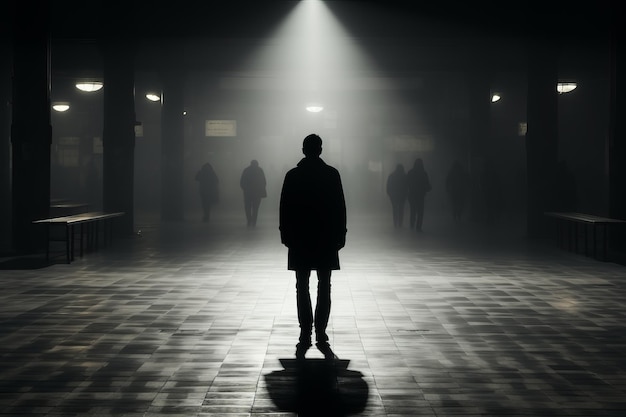In this black-and-white photograph, a lone man stands in the center of a dimly lit room, his tall silhouette illuminated by a spotlight overhead that casts a distinct V pattern of light down his body. He wears a long coat, and his features are obscured by shadow, although the back of his head is clearly visible. The man appears to be standing on tiptoes on a tiled floor, which also reflects his shadow. Surrounding him in the background are the indistinct shadows of five figures, moving towards him but lacking any identifiable facial details. The scene is set within a large building or likely a basement, evidenced by the presence of multiple pillars that provide some structure in the otherwise shadowy space. The composition of the image emphasizes the isolation of the central figure, highlighted starkly against the vague forms approaching him.